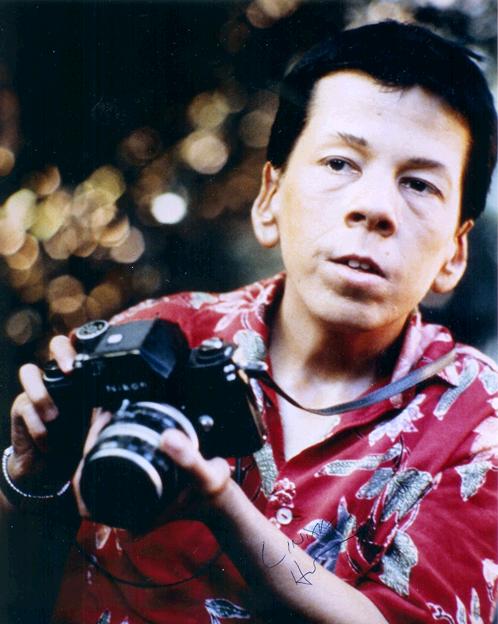This image is a color photograph of a middle-aged Asian man holding a camera, appearing ready to take a photo. He has very dark hair and distinctive ears that stand out a bit. The man is wearing a short-sleeve red Hawaiian shirt adorned with blue and white flowers, suggesting it might be a hot day. His right hand is poised over the shutter button while his left hand supports the camera's larger lens. A camera strap encircles his neck. The background is blurred and presents a mix of darker tones that cannot be clearly identified. There is a signature at the bottom of the image, but it is too obscure to read clearly. The focus is clearly on the man as he prepares to capture a photo.